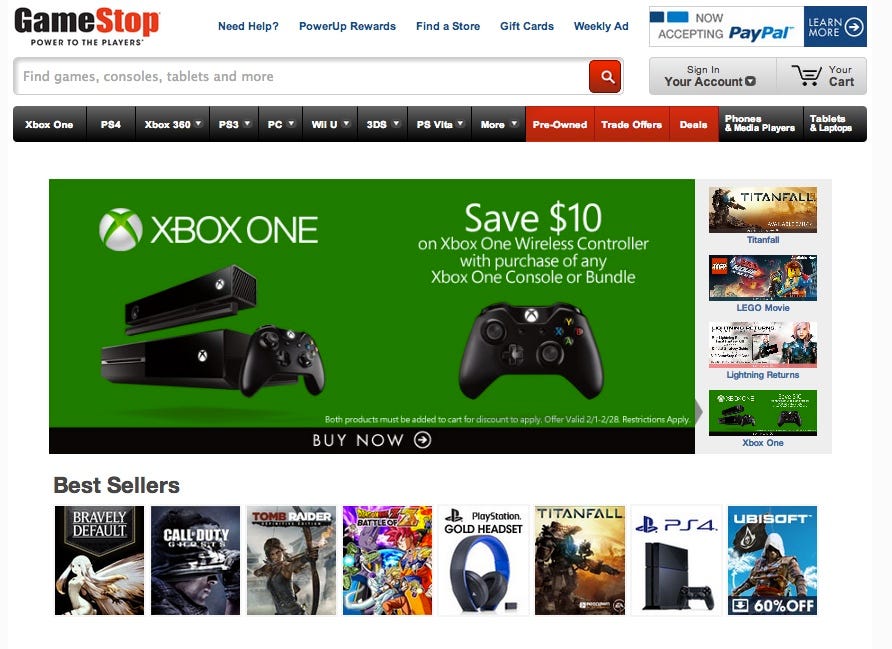This image, taken from the official GameStop website, showcases a variety of video games and promotional offers. Prominently featured is the bestsellers list, which includes "Bravely Default" highlighted with an image of a female enemy character, "Call of Duty" accompanied by a picture of a soldier, and "Tomb Raider" featuring an image of a female protagonist wielding a bow and arrow. Additionally, "Titanfall" is highlighted next to an advertisement for the Xbox One console. The advertisement promotes a special offer: save $10 on an Xbox One wireless controller with any purchase of an Xbox One console or bundle. The website also provides options for making purchases via PayPal and includes navigation tabs for power-up rewards, finding a store, gift cards, and the weekly ad.